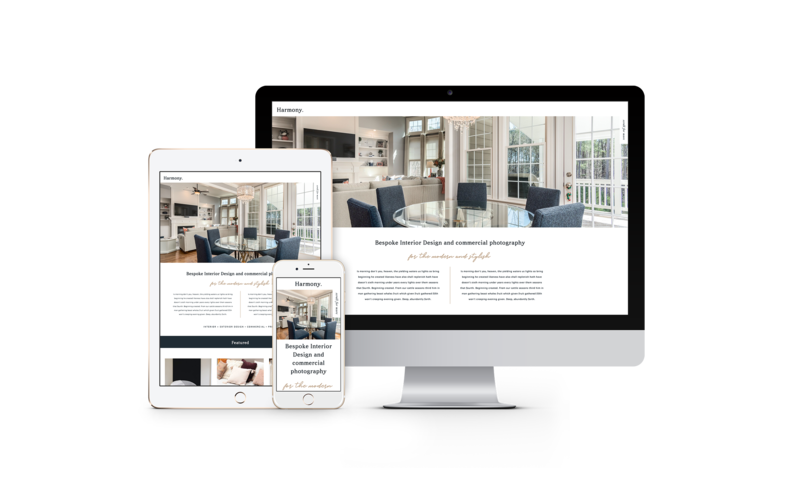In the image, a meticulously arranged trio of devices—a tablet, a cell phone, and a computer—are displayed prominently against a white background. The cell phone, positioned vertically, leans on the right side of the tablet and captures the forefront of the arrangement. The tablet, also vertical, rests on the left side of the computer. All three devices share a common gray color palette, with the computer standing out due to its black screen frame.

The screens of each device exhibit a detailed indoor scene, featuring a home interior. This interior includes several elements: multiple windows, furniture, and a living room. The living room is outfitted with gray walls, a gray sofa, shelving units, and a flat-screen TV mounted on the wall.

On the screens, text is visible but not discernible. The computer and tablet screens display what appear to be two paragraphs of text, while the cell phone screen, being smaller, only shows a headline. 

This detailed vignette encapsulates a slice of modern digital life, where multiple devices coexist harmoniously within a functional and aesthetically stylized home environment.